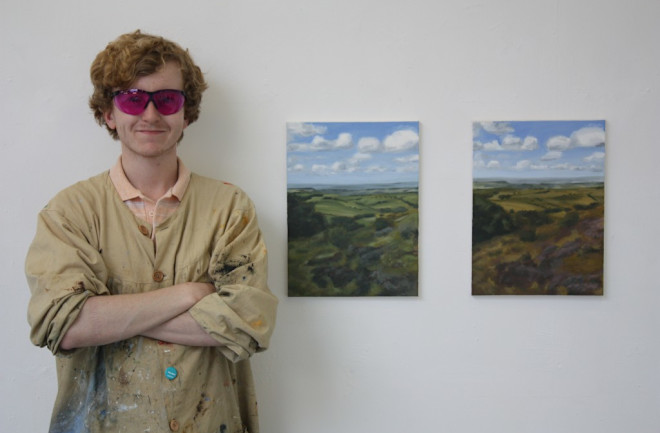The image features a young Caucasian man standing in front of a soft gray background, beside two aerial landscape paintings. The paintings depict the same scene with varying color schemes, possibly representing different seasons—one characterized by rich greens and the other by browns. Each artwork captures a panoramic view of canyons, trees, fields, and mountains under a blue sky adorned with cloud structures at the top.

The young man is proudly smiling, wearing distinct pink-tinted sunglasses, and exudes an artistic aura. He is dressed in a well-worn, paint-splattered beige smock over an apricot-colored polo shirt. His auburn hair is relatively short, and his face shows signs of casual grooming. He stands with his arms folded, displaying part of his forearms. Behind him, the white wall provides a neutral backdrop that accentuates both his presence and his artwork.